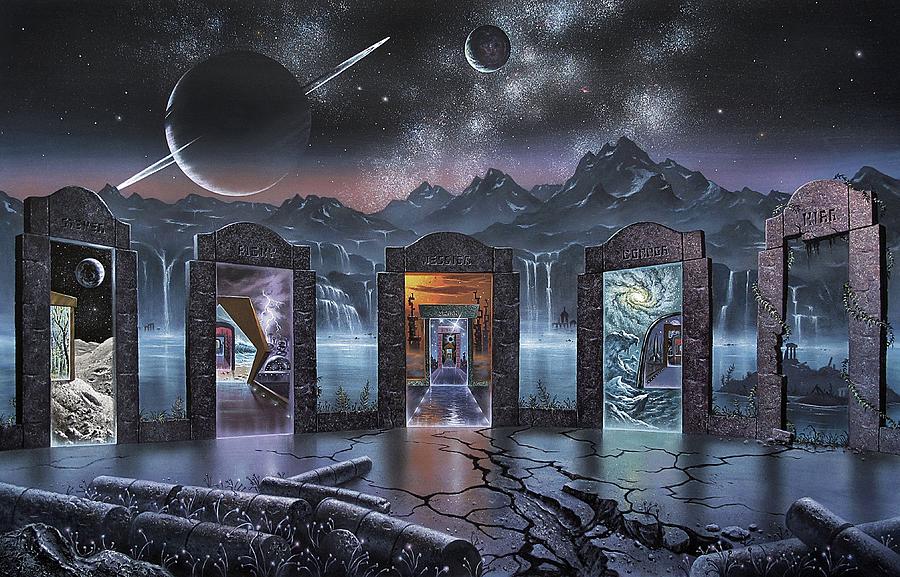In this detailed and evocative computer-generated illustration, we find ourselves at the edge of a cracked, black platform that appears to hover over a dark expanse of water. The scene is drenched in ominous, shadowy hues, emphasizing the dark nature of this fantastical landscape. Before us, five enigmatic portals or doorways span in a slight curve, each radiating an aura of mystery and adventure.

The central doorway leads through an orange-lit pathway to another enigmatic threshold, perhaps indicating a further journey within. To its immediate right, the fourth portal swirls with a cosmic nebula, evoking a sense of boundless space and time. The farthest right doorway, shrouded in darkness, seems to offer a direct glimpse into the distant, jagged mountains that loom behind the portals, cascading with numerous waterfalls feeding into the immediate watery foreground.

On the left side, the first portal reveals a celestial landscape under a moonlit sky, perhaps another world bathed in silvery light. The second doorway crackles with a flash of lightning over an obscure, tumultuous horizon reminiscent of a stormy beachscape. All portals are surmounted by curved, ornate arches inscribed with unreadable, otherworldly hieroglyphics, adding to the arcane atmosphere.

Behind these portals, the scenery unfolds into an impressive backdrop of dark, craggy mountainsides, heavily dotted with waterfalls that disappear into the expansive body of water. Above these mountains, the sky is an ethereal, cosmic interlude filled with impending celestial bodies; a dark, ominous planet resembling Saturn, with its distinctive rings, looms large, while another unidentifiable orb hovers just beyond. Spray-painted clouds and twinkling stars add to the surreal, almost painted quality of the skyscape.

Scattered across the fractured surface of the platform are cylindrical objects, seemingly metallic and askew, contributing to the scene's otherworldly and futuristic nuance, as though they were remnants of an ancient, abandoned technology. This dark yet intricately detailed illustration could easily be a still from a science fiction movie or a high-fantasy video game, inviting viewers to ponder which of the five enigmatic portals they would choose to step through into another realm.